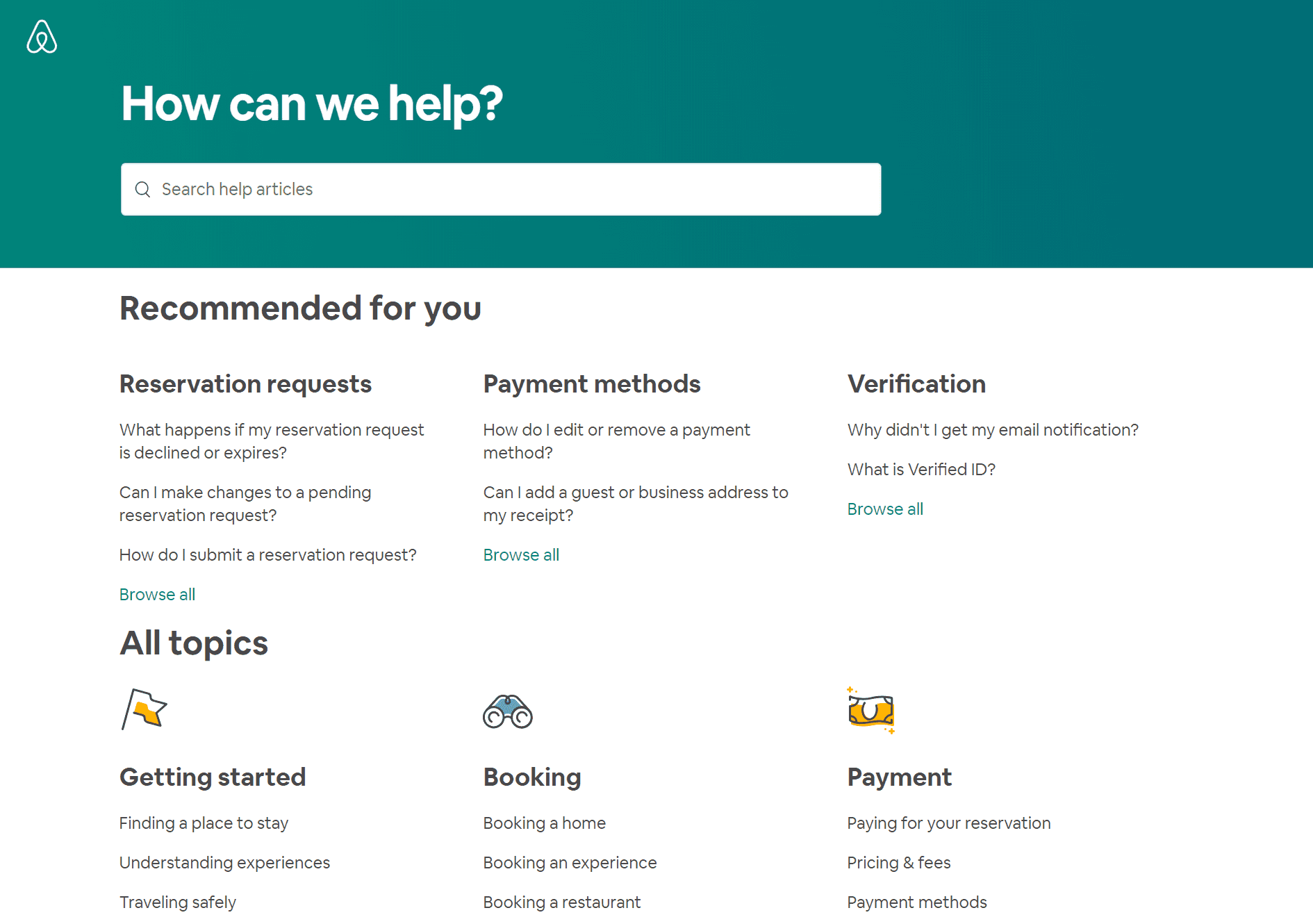### Descriptive Caption:

The upper portion of the image features an aqua rectangular box with a white logo in the top left corner. To the right of the logo, bold white text reads, "How can we help?". Below this, a horizontal rounded rectangle contains light grey text, "Search help articles," accompanied by a light grey magnifying glass icon on the left.

Beneath this section is a white background displaying various texts. Directly under the search bar, in bold black text, it says, "Recommended for you." This section is divided into three columns. The first column is titled "Reservation Requests," the second "Payment Methods," and the third "Verification."

Under "Reservation Requests," several questions are listed:
- "What happens if my reservation request is declined or expires?"
- "Can I make changes to a pending reservation request?"
- "How do I submit a reservation request?"

There is also a blue text link that says, "Browse all."

Further down, another bold black headline reads, "All topics." Beneath this, there are various sections with associated icons and text:
- An image of a white and orange flag next to the text, "Getting started."
- An image of a book next to the text, "Booking."
- An emoji of a dollar sign next to the text, "Payment."

Under each of these sections, additional relevant black text is displayed.